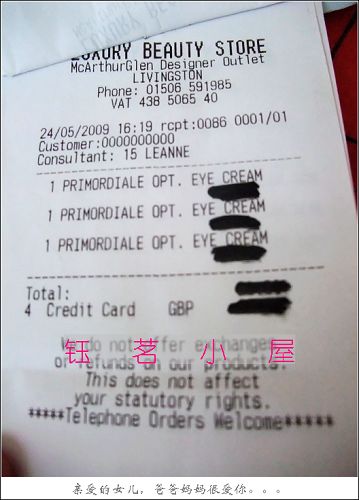The image depicts a white receipt with black printed text. It is from "Luxury Beauty Shop" located at MacArthur Glen Designer Outlet in Livingston. The phone number listed is 015-06-59-1985 and a reference number reads 438-5065-40. The receipt is dated 24th May 2009 at 16:19 and is identified as receipt number 0086-0001-01. The customer ID is filled with zeros, and the consultant ID is 15, named Leanne. The purchased item, "Primordial Opt Eye Cream," is listed three times. The total amount, paid by credit card, has been blacked out with a marker. Additionally, the bottom of the receipt features some information overlaid with pink characters, written in what appears to be Chinese or another Asian language.